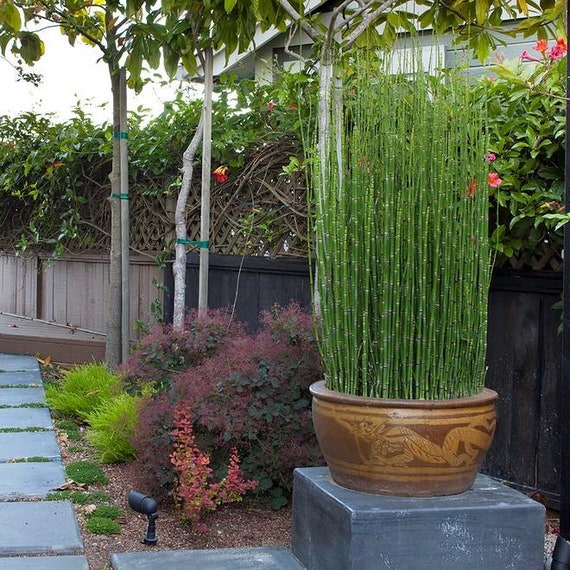The image captures a small, meticulously manicured backyard garden, bordered by a black fence that supports climbing plants. Beyond the fence, a neighbor's light blue house with white eaves is visible. The garden features large, rectangular paving stones set into the dirt, creating a structured pathway. Various shrubs and colorful plants, exhibiting shades of green, dark green, and maroon, enhance the garden's vibrancy.

In the foreground, cement steps lead to multiple platforms. Atop the tallest platform rests an old-fashioned, ornate pot, which appears to be made of wood and carved with a dragon motif. This pot contains hundreds of uniformly tall, thin bamboo shoots, tightly clustered together like straws in a box. Below this pot are two distinct plants, contributing additional hues to the scene. A directional light fixture is embedded in the ground to provide ample illumination at night. The overall composition of plants, stonework, and decorative elements create a lush and inviting atmosphere in this quaint backyard.